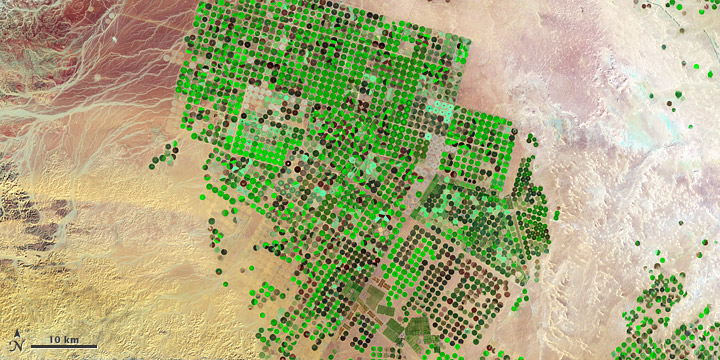The image is a horizontally rectangular, multi-colored map or satellite image, devoid of borders or a specific background. In the lower left-hand corner, there is black text showing the letter "N" with an arrow pointing upwards, next to a vertical black line. Above this line, "10 km" is written, presumably indicating kilometers. The left side of the image is dominated by reds, pinks, and yellows, interspersed with vein-like white lines. The center features clusters of green, brown, and black circles, arranged in rows and grids, forming various rectangles and squares. The upper right and lower right corners display these circles as well, although they are sparser compared to the center. The colors transition to a lighter palette of purple, pink, and white. The dots might be military markings or targets, with some of them appearing darker in hue, hinting at possibly strategic points or special significance.